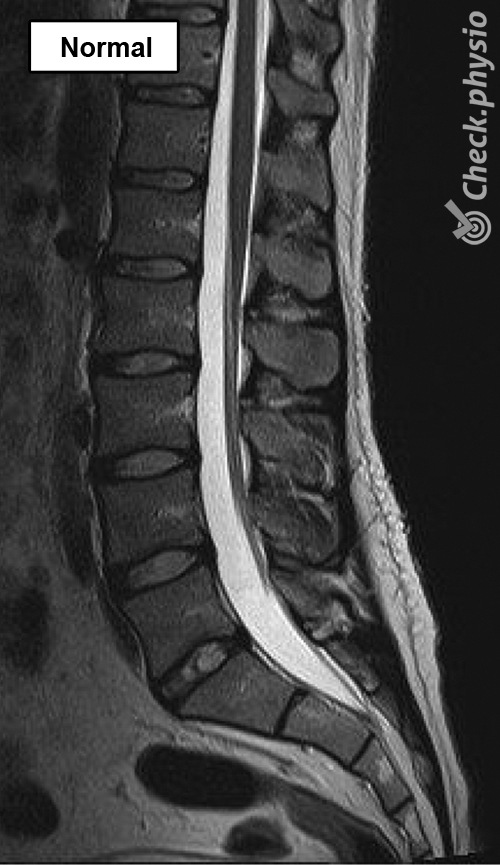The black-and-white image appears to be an x-ray scan of the lower spine, displaying a profile view. The majority of the spine is depicted vertically with a slight curve near the tailbone at the bottom right. In between the large vertebral bones, small gaps are visible. Adjacent to the spine, a prominent white line runs the length of the image, which could be part of the scan or a calibration marker. The x-ray details skin, muscle, and possibly fatty tissue structures around the spine. The background of the image is predominantly black.

In the top left corner of the image, there's a white rectangle featuring the word "normal" in black text, indicating that the scan shows a healthy spine. On the right side, written sideways and upside-down, there's a logo with a checkmark inside a bullseye next to the text "check.physio," likely referencing that the x-ray was reviewed or authorized by a physiologist.